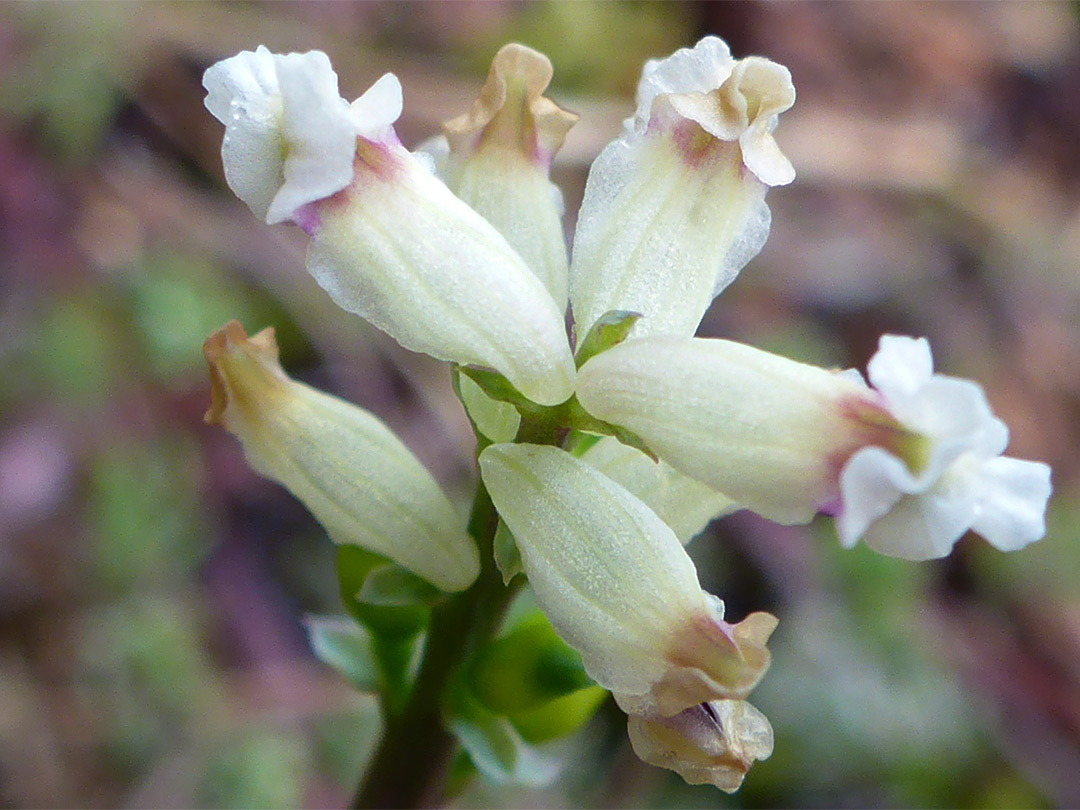This photograph, taken outdoors during the daytime, is a close-up of a partially bloomed flower head, centrally framed in a horizontally aligned rectangular image measuring approximately six inches wide by four inches high. The focus is on a cluster of elongated, trumpet-shaped white blooms, each tinged with subtle hues of purple, pink, green, and beige at the frilly ends where the petals start to open. There are about seven of these tubular blossoms, radiating outward in various directions – three to the left, two to the right, and two behind them. Some of the blooms show signs of wilting, with brown tips contrasting against the predominantly white petals. Below the flowers, a sturdy stem, transitioning from reddish at its base to green towards the top, supports the blooms and bears tiny green leaves. The stem slants slightly to the right. The background is artistically blurred, filled with soft blends of green, purple, and white tones, suggesting the presence of more flowers and natural elements, likely a forest floor with ivy and leaf litter.